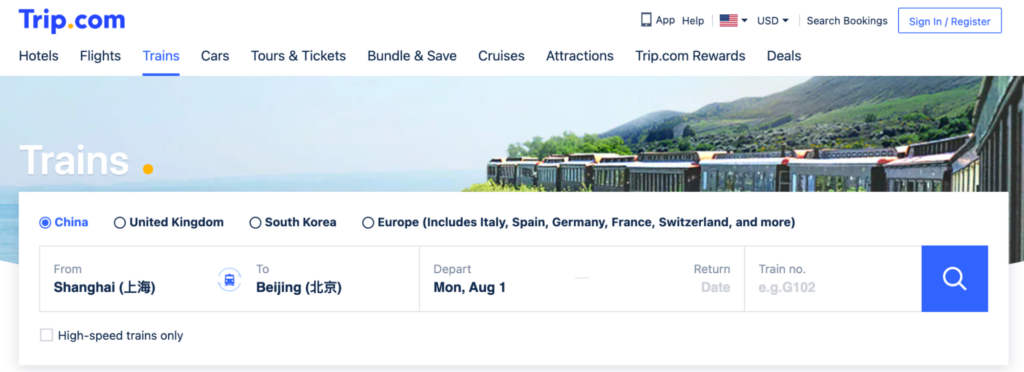The image captures a webpage from trip.com. At the top of the page, the website's name "trip.com" is prominently displayed in blue, with the dot in yellow. The navigation menu includes clickable sections such as Hotels, Flights & Trains, Cars, Tours & Tickets, Bundle & Save, Cruises, Attractions, trip.com Rewards, and Deals. Additional options at the top include "App," "Help," an American flag icon indicating the language/currency set to USD (with a dropdown menu), a search bookings feature, and a "Sign In/Register" button within a highlighted box.

The image highlights that the "Trains" section has been selected, evident from its blue color and accompanying yellow dot, distinguishing it from the other black-colored options. Below this, regional options are presented, and the user has selected "China." Other selectable regions include the United Kingdom, South Korea, and various European countries such as Italy, Spain, Germany, France, Switzerland, among others.

Further details show that the chosen train route is from Shanghai to Beijing, with the travel date set for Monday, August 1st.